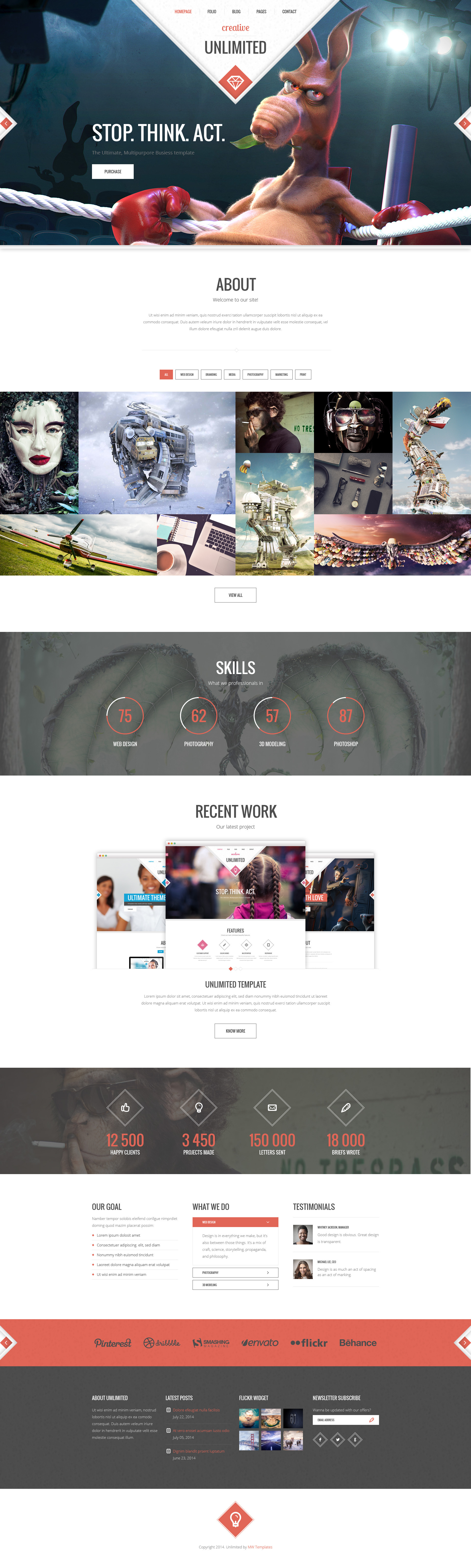The image is a detailed screenshot of a vibrant web page. At the top, a cartoon kangaroo is depicted in a boxing ring, leaning against the white ropes. The kangaroo is wearing red boxing gloves and is positioned under the statement "Stop, Think, Act," which is written in bold, white font. Illuminating lights create a dramatic background behind the kangaroo. Below this, a white banner with the word "Unlimited" accompanied by a down arrow is prominently featured. The web page includes an "About" section.

Colorful advertisements fill the page, including an image of a geisha-like woman with a white face and red lips, and a robot suspended in mid-air. Additionally, images of a chimpanzee and a futuristic AI-type robot are present. The page displays various skill indicators, each represented by numbers in red circles. A "Recent Work" section is also visible, showcasing different achievements. At the bottom, diamond shapes contain numbers: 12,500, 3,450, 150,000, and 18,000, presumably representing some form of statistics or milestones.